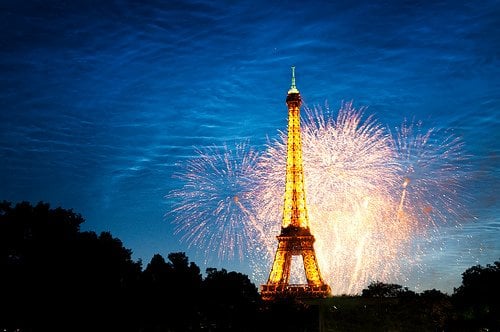This photograph captures a stunning evening celebration centered around the Eiffel Tower, which is bathed in a majestic golden light. The sky, transitioning from dark blue to lighter blue with rippling cloud patterns, provides a dramatic backdrop. Dominating the scene, the Eiffel Tower stands slightly to the right of the center, glowing brightly. Surrounding it, a spectacular display of fireworks bursts into the sky, featuring vibrant hues of red, yellow, and orange. These fireworks, some almost as tall as the Eiffel Tower itself, illuminate the scene with festive energy. The foreground is silhouetted by darkened trees, emphasizing the nighttime ambiance. The overall composition creates an enchanting and vivid portrayal of a celebratory evening in Paris.